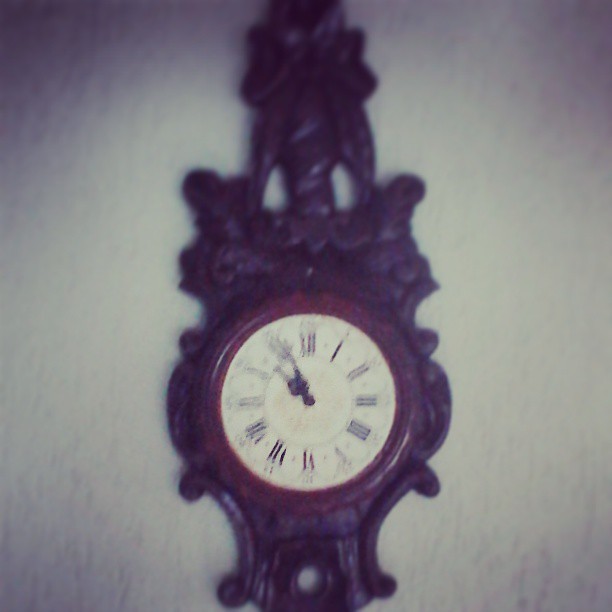The photograph is a blurry, color image of an antique wooden clock hanging on a white wall. The clock's casing is brown wood, adorned with intricate swirly filigree engravings above and below the white clock face. At the top of the clock, there is a long, tapering shape, possibly a bow, although the blurriness makes it difficult to discern specific details. The clock face features Roman numerals in an old English style to mark the hours. The hour hand is pointing between the numbers X (10) and XI (11), while the minute hand is pointing directly at XI (11), indicating the time is approximately 10:55. Despite its complex design, no clock hands are connected to any bands, and the visible holes at the bottom confirm the absence of these features.